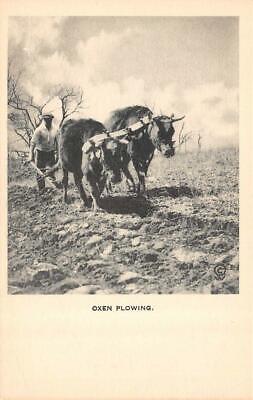The image, presumably scanned from an old photograph, appears on the sepia-toned, yellowing page of possibly a vintage textbook or document. The black-and-white photograph, centrally placed and slightly elevated on the page, features two oxen yoked together, plowing a barren, rocky dirt field. A farmer, dressed in a shirt and what appears to be a tank top, follows them, holding the wooden handle of the plow. Sparse, dry trees dot the distant landscape under an overcast sky, the clouds dulling any potential brightness. The photograph, marked by heavy compression and noticeable JPEG artifacting, shows the oxen tirelessly at work in the expansive field, evoking a sense of historical agricultural practices. Below the image, the text reads "Oxen plowing," succinctly summarizing the scene. The photograph occupies about three quarters of the vertical rectangle of the sepia page, with the rest of the page serving as a muted backdrop to this poignant agricultural tableau.